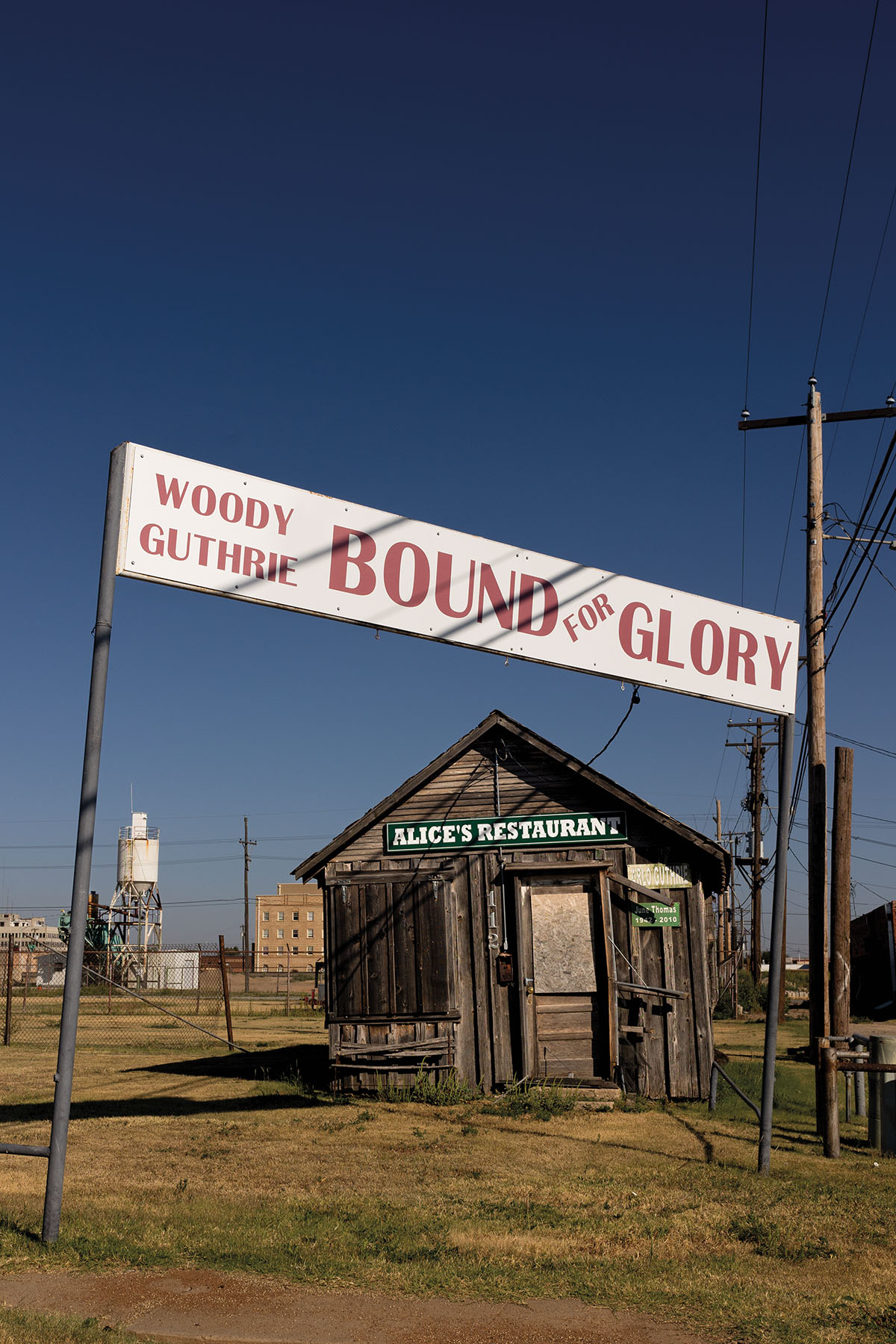In this daytime nature image, there's a dilapidated, small wooden building that appears to be an old restaurant or shack with a sign that reads "Alice's Restaurant" in green. The structure is dark and weathered, with boarded-up windows and door, hinting at a once-thriving establishment now in disrepair. In the foreground, there's yellowed grass, indicating a lack of upkeep or drought conditions. Staked into the grass is a white sign with red lettering that reads "Woody Guthrie Bound for Glory," held up by two poles. The scene is devoid of people and major objects, giving it an abandoned, almost ghost-town feel. The background features a larger building, telephone wires, and possibly white and silver machinery or factory equipment. The sky above is a deep blue, pointing to a clear, sunny day despite the overcast atmosphere of neglect and abandonment. The image’s color palette includes neutrals punctuated by green, yellow, blue, and red.